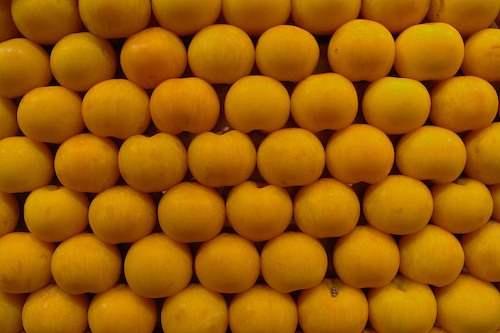This close-up photograph showcases a tightly packed arrangement of small, round fruits, most likely yellow apples, though their orangey-yellow hue has led to some debate. Captured from an indeterminate angle, the apples fill the frame, their slight dimples and occasional stems visible among them. With at least seven rows and approximately seven columns, there are around 49 apples in view, forming a near honeycomb-like structure due to the snug spacing. The lighting—dim and seemingly from above—casts a light shadow, adding depth to the image. The lack of context leaves it unclear whether the apples are in a basket, on a shelf, or part of a display. A tiny bumblebee can be seen resting on an apple towards the bottom row, adding a subtle detail to the overall composition.